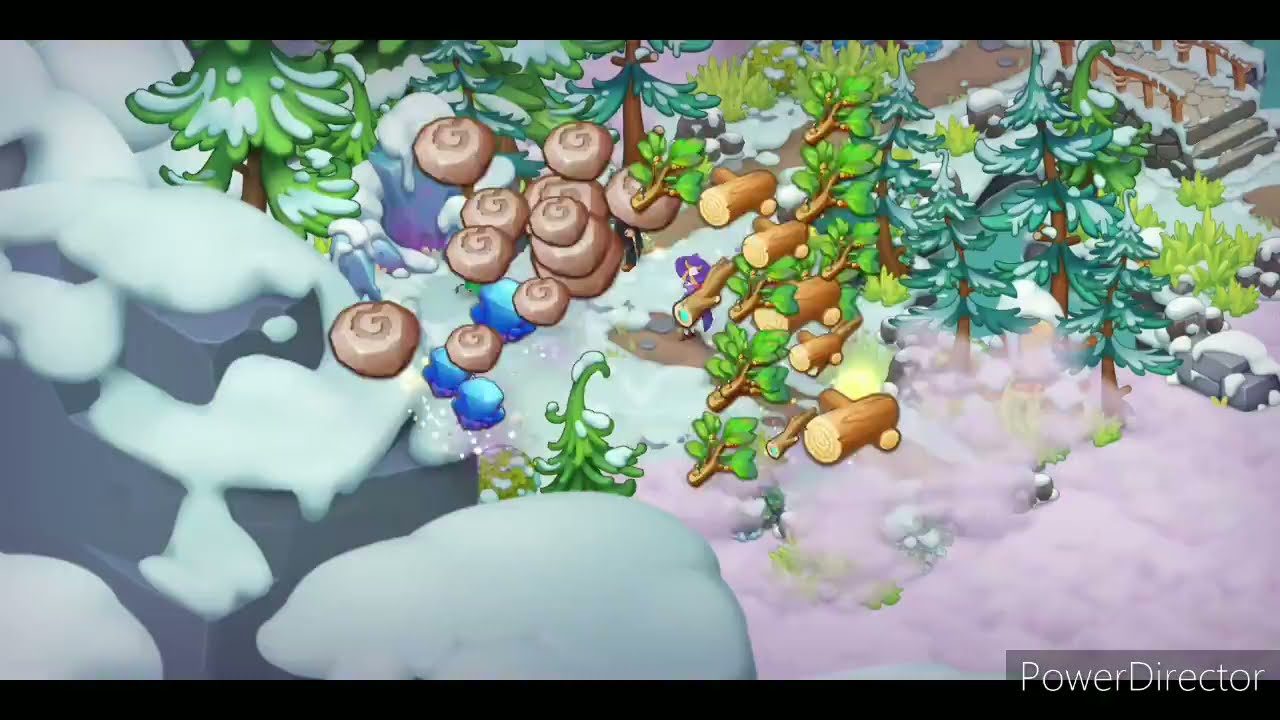This image is a detailed screenshot from an animated computer or mobile game, depicting a cartoonish top-down view of a snowy landscape. On the left side, large gray stones are covered in snow, possibly bordering a cliff or slope. The center and right of the image feature snow-laden cartoon trees, sparsely populating the snowy forest floor. Scattered across the scene are several overlapping cartoon symbols including green-leafed branches, large sawed-off logs, precious-looking blue rocks, and light brown circular stones adorned with swirly patterns. Near the center of the image, a partially obscured character with purple hair can be discerned amidst the items. Additionally, a visible path or staircase can be seen towards the top right. The lower right corner contains text reading "Power Director."